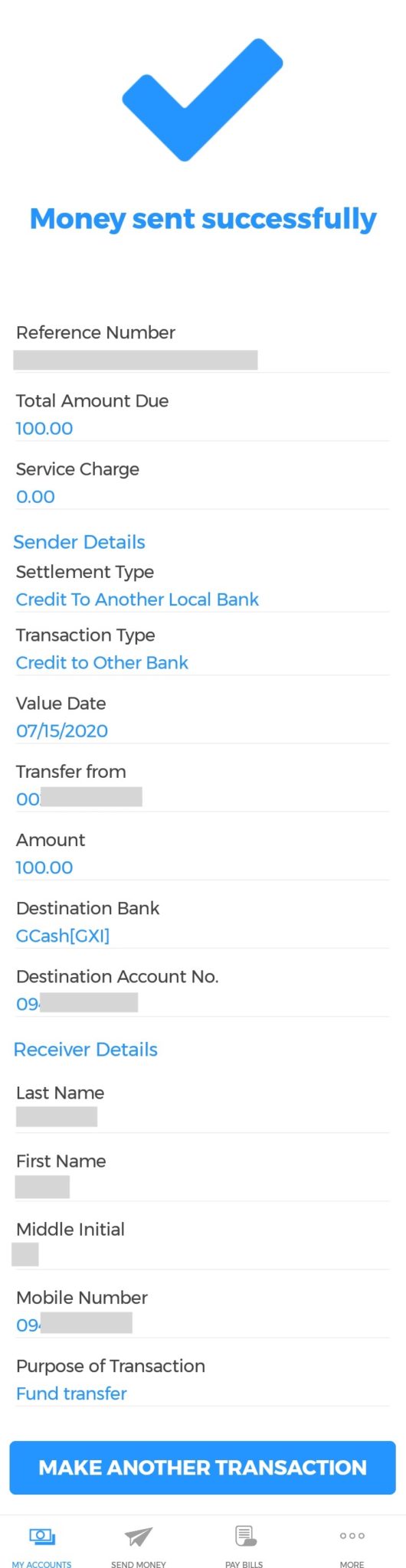This image depicts a webpage from a money transfer service, showcasing the successful completion of a transaction. At the very top, a blue check mark is prominently displayed, followed by the message "Money Sent Successfully" in blue text. Directly below, in black text, is the "Reference Number," accompanied by a gray bar likely containing the actual reference number.

Continuing downward, the left side of the screen displays relevant transaction details in black text. It starts with "Total Amount Due," paired with the amount "$100" in blue text. Next, "Service Charge" appears in black, with a corresponding value of "Zero" in blue. 

Further details include "Sender Details" in blue, followed by the "Settlement Type" described as "Credit to another local bank" in black text. Similarly, "Transaction Type" is listed as "Credit to other bank". The "Value Date" marked "07-15-2020" appears with a redundant second mention of "Value Date" directly below it.

The section "Transfer From" has its information obscured, while the "Amount" is confirmed as "$100." A gray line separates these from the "Destination Bank," which is listed as "See Cash," and the "Destination Account Number," which is also blocked out.

At the bottom of the page, "Receiver Details" is indicated, requesting the receiver's last name, first name, middle name, and mobile number.